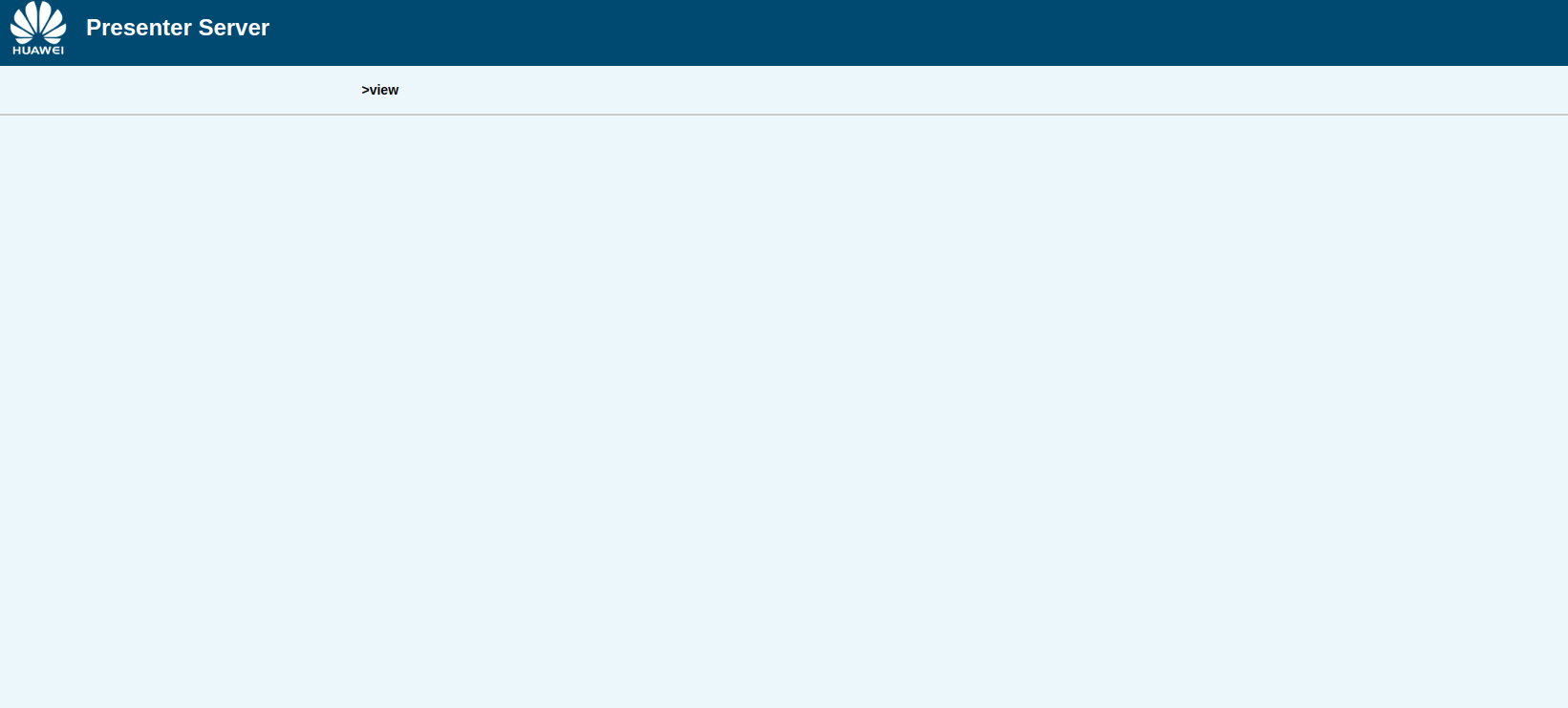This is a screenshot of a Huawei mobile company website. The page is largely blank, with only a minimal top header providing information. The header, colored navy blue, features the Huawei logo on the far left. The logo resembles radiating white flower petals. Adjacent to the logo, in white text, are the words "Presenter Server." Below this, there is a smaller line of text in black that reads "View," accompanied by a small arrow pointing to the word. Underneath "View," a horizontal border is visible. The web page itself has a very light blue background and remains otherwise blank, with no additional content loading.